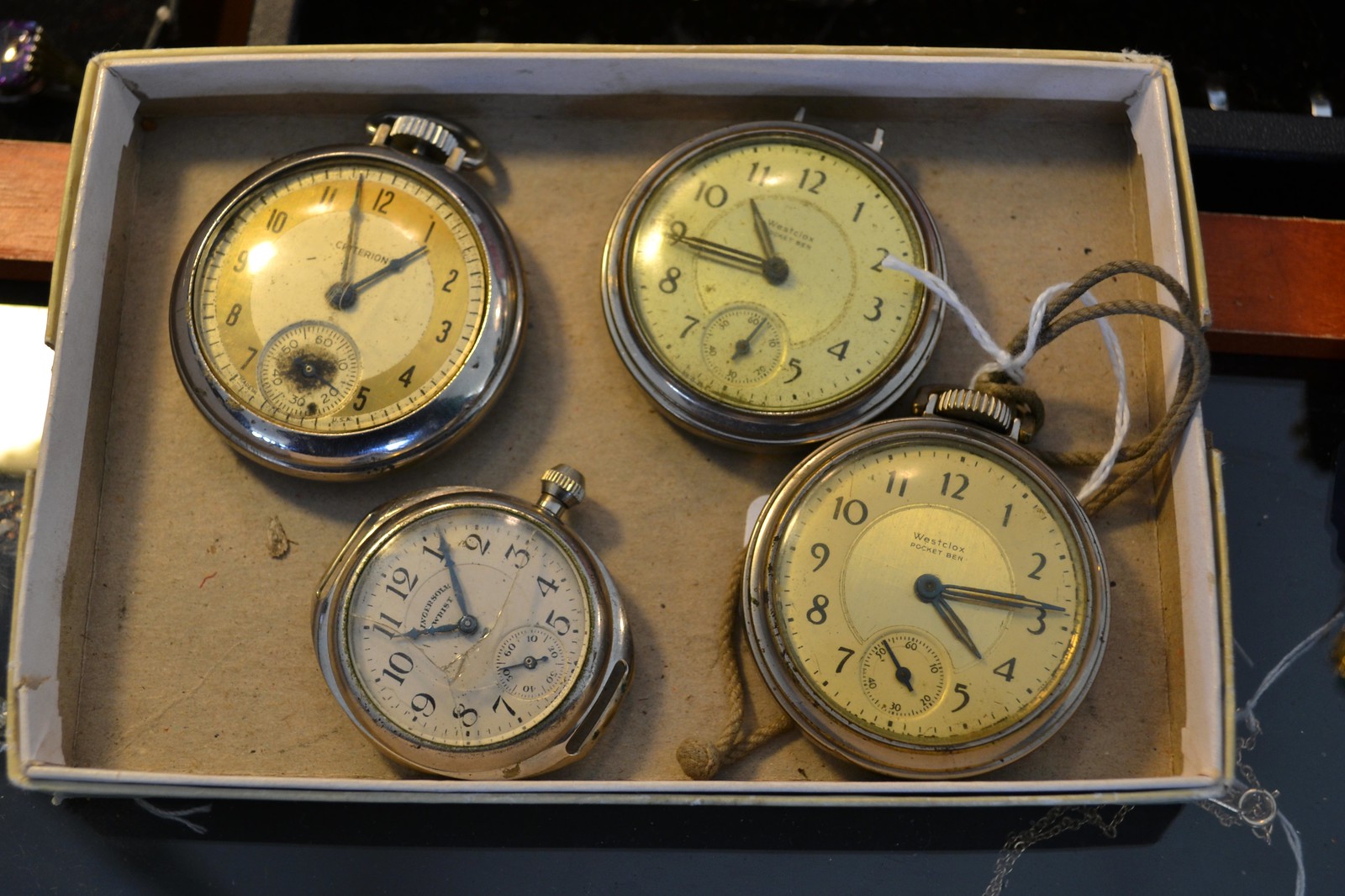This overhead photograph features a close-up view of four antique pocket watches neatly arranged in a shallow, light brown cardboard box, likely a repurposed puzzle box. The box dominates the frame, leaving the surrounding environment indistinct. The pocket watches are organized in two rows of two. Three watches, with open faces and simple black numerals and notches, exhibit a faded yellow patina on their faces, indicative of their age. These timepieces, metallic silver and roughly hand-sized, have small black hands, and two of them show different times, such as 11:11 and 4:14. The fourth watch in the bottom left corner stands out due to its smaller size and noticeably whiter face, suggesting it is relatively newer. Additionally, the watch in the lower right corner has a piece of brownish yarn or cloth string attached to it, adding a touch of rustic charm to this collection of historic timekeepers.